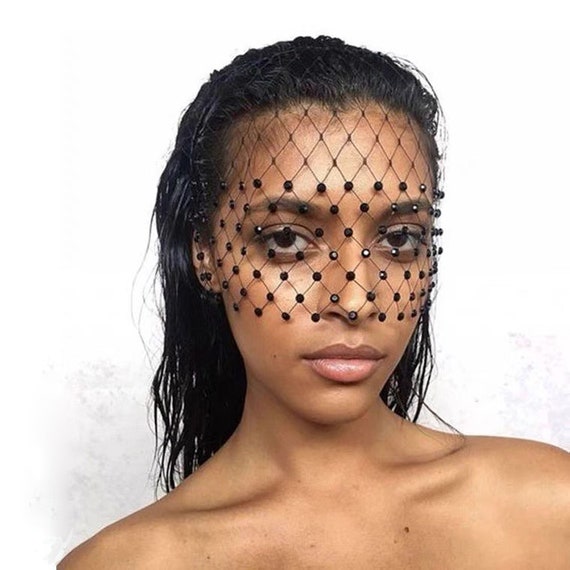This is a vertical rectangular photograph of a woman with dark brown skin and black hair that falls just below her shoulders, appearing to be either straightened or wet. She is wearing a black veil that drapes over the top of her head and covers from her forehead down to the tip of her nose. The veil features a diamond-shaped pattern with prominent black spots or beads at the junctions of each diamond, obscuring her eyes as she looks through this mesh. Her big brown eyes have a slightly lazy, bored expression as she stares directly into the camera. The background is a very light gray to white, giving no additional context. The woman’s bare shoulders and collarbone are clearly visible, indicating she is not wearing any clothing on her upper body.